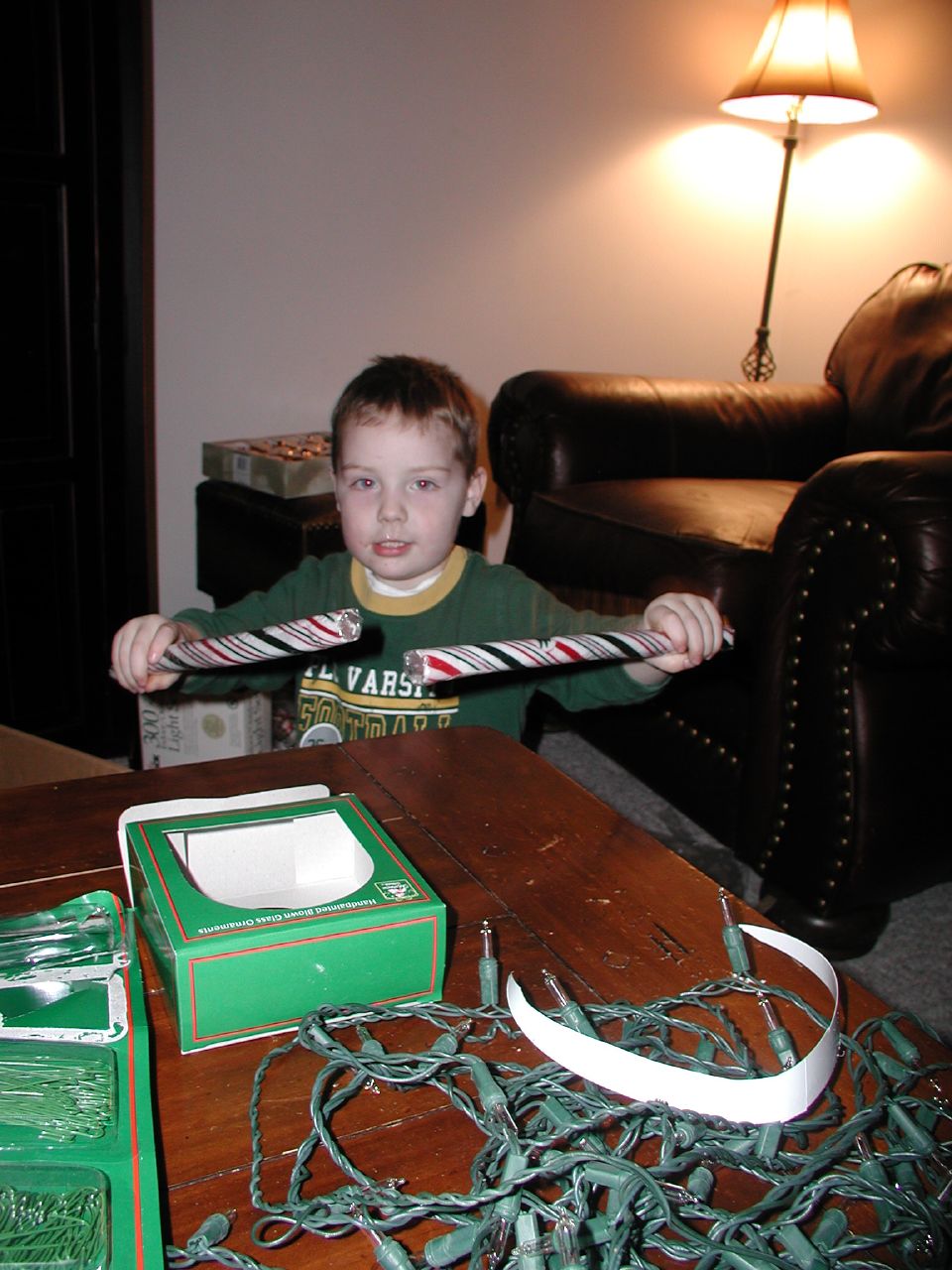In this festive photo taken around Christmas, a young boy, approximately 4 or 5 years old, stands behind a large dark wooden table in what appears to be a living room. The boy, who has short ash-blonde hair, is wearing a green crewneck sweater with white lettering that reads "Varsity," although only the letters "V-A-R-S" are clearly visible. The sweater features a distinctive honey mustard-colored collar. The boy is looking directly at the camera, holding two rolls of wrapping paper with red and blue stripes, each hand gripping one roll with the edges pointed towards each other.

In front of him, the table is cluttered with various Christmas decorations. A heap of green Christmas lights lie tangled on the table's surface, seemingly spilled from an open green box nearby. To the left, there's another container, possibly holding small wire hooks or clips used to attach ornaments, adorned with a red stripe. 

In the room's background, a cozy scene unfolds: a tall lamp is lit, casting a warm glow, and a one-seater leather chair is visible next to a dark brown doorway. An ottoman nearby has some indistinct items on it, potentially more Christmas decorations. The white wall behind adds to the festive yet homely atmosphere captured by the photo.